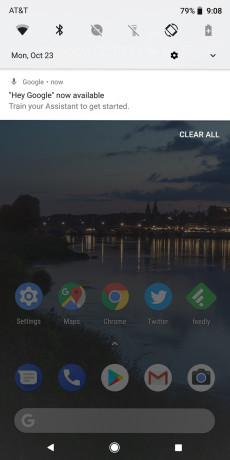This image depicts a smartphone display. The status bar at the top shows AT&T as the carrier, along with icons for Wi-Fi and Bluetooth (currently active), a flashlight and another feature that appear to be disabled, and a battery meter indicating 79% remaining battery life. The time reads 9:08, and the date below is Monday, October 23rd. There is also a settings gear icon and a downward-pointing arrow nearby.

Below the status bar, the screen displays a notification promoting Google Assistant, which reads, "Hey Google now available. Train your system to get started." In the top right corner, there's an option to "Clear All" notifications. The device's wallpaper appears to be a tranquil evening scene at a marina, with boats docked and lights reflecting off the water, suggesting it's around dusk.

The homescreen is organized neatly with two rows of five icons each. The top row features: 
1. Settings (white gear icon)
2. Google Maps
3. Google Chrome
4. Twitter
5. Feedly (a green icon that looks like a diamond with white lines).

The second row includes:
1. Messages (chat bubble icon)
2. Phone (handset icon)
3. Google Play Store
4. Gmail
5. Camera (camera icon).

At the bottom of the screen is a Google search bar for quick access to searches.